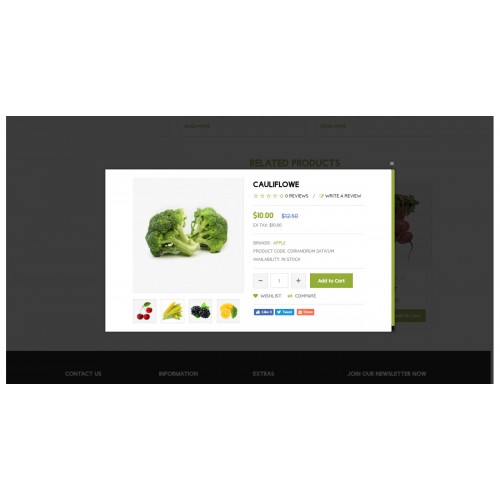The pop-up displayed on the grey-layered website is predominantly white and obstructs most of the content behind it. In the top right corner of the pop-up, there is an "X" button for closing the window. The heading of the pop-up reads "cauliflower," though it is misspelled as "C-A-U-L-I-F-L-O-W-E." There are no reviews available, and the price is listed as $10. Due to poor resolution, the text is difficult to read, making details like tax information illegible.

Within the pop-up, there is an image of a cauliflower prominently featured. Below this main image, there are four smaller pictures showing cherries, corn, blackberries, and lemons. The images have poor readability, and there's an indication that an item is being added to the cart, although the specifics are unclear. There is also a reference to "apple" and something labeled "perfect cocoa," but these details cannot be deciphered due to the low resolution.

Social media interaction options are present, including a Facebook "like" button, a tweet button, and an orange button that is likely for Reddit. The images themselves display vibrant colors: a green cauliflower, red cherries, yellow and green corn, green and black blackberries, and yellow and green lemons.